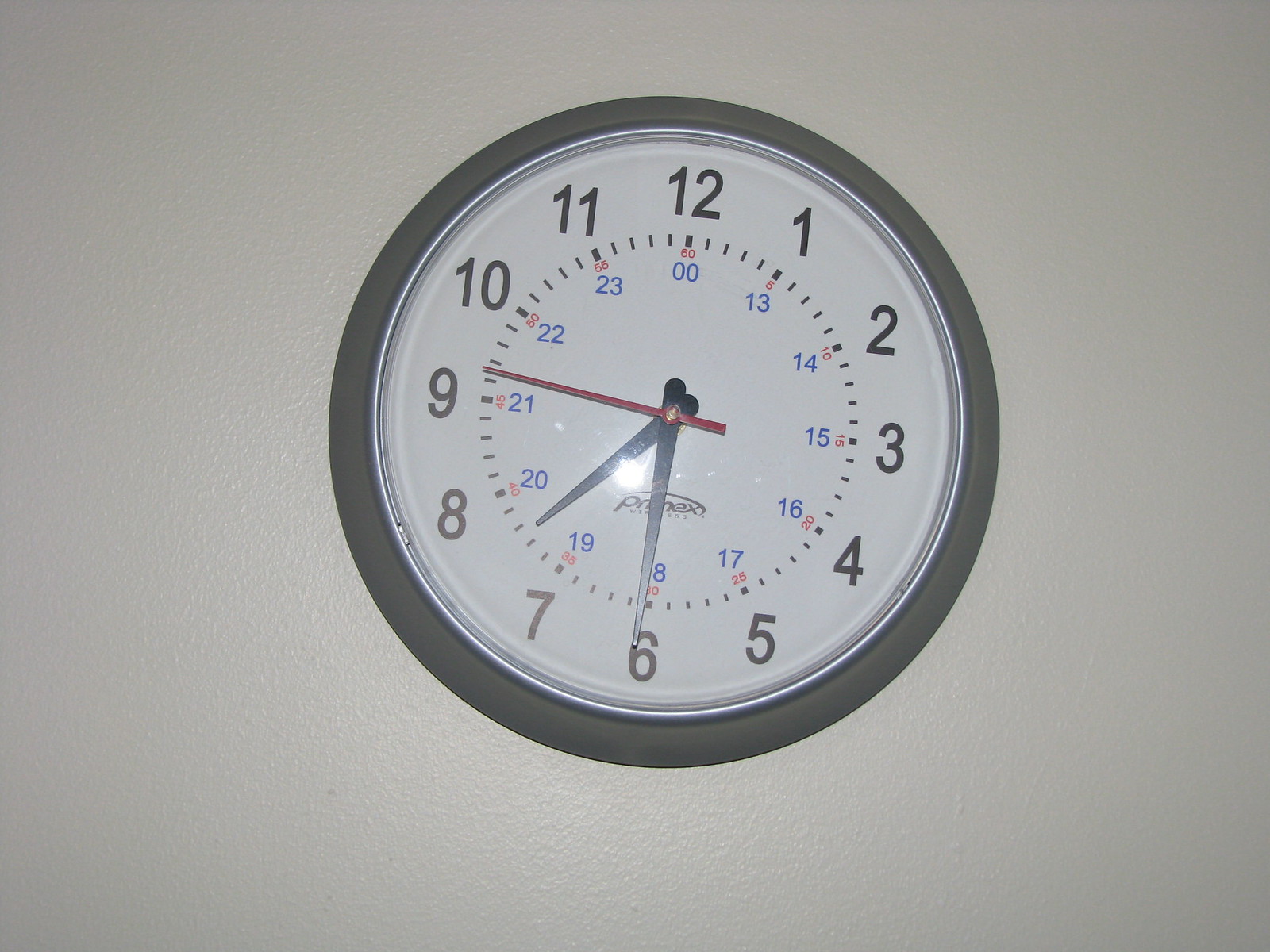The photograph depicts a wall clock hanging on an off-white wall, slightly tilted with the 6 offset to the left and the 12 to the right. The clock's frame is black with a clear, likely plastic, protective cover. The face is white, featuring large black numbers for the hours, numbered 1 to 12, and three distinct sets of additional numbers. The smallest inner numbers, in blue, indicate the 24-hour time from 00 to 23. Surrounding these, in red, are the minute and second markers, going from 5 to 60 in increments of five. The outermost edge displays black numbers for the standard 1 to 12-hour time. The clock shows the time as 7:31 and 47 seconds, with a long, thin red second hand, a black minute hand pointing at the 6, and a shorter black hour hand past the 7.